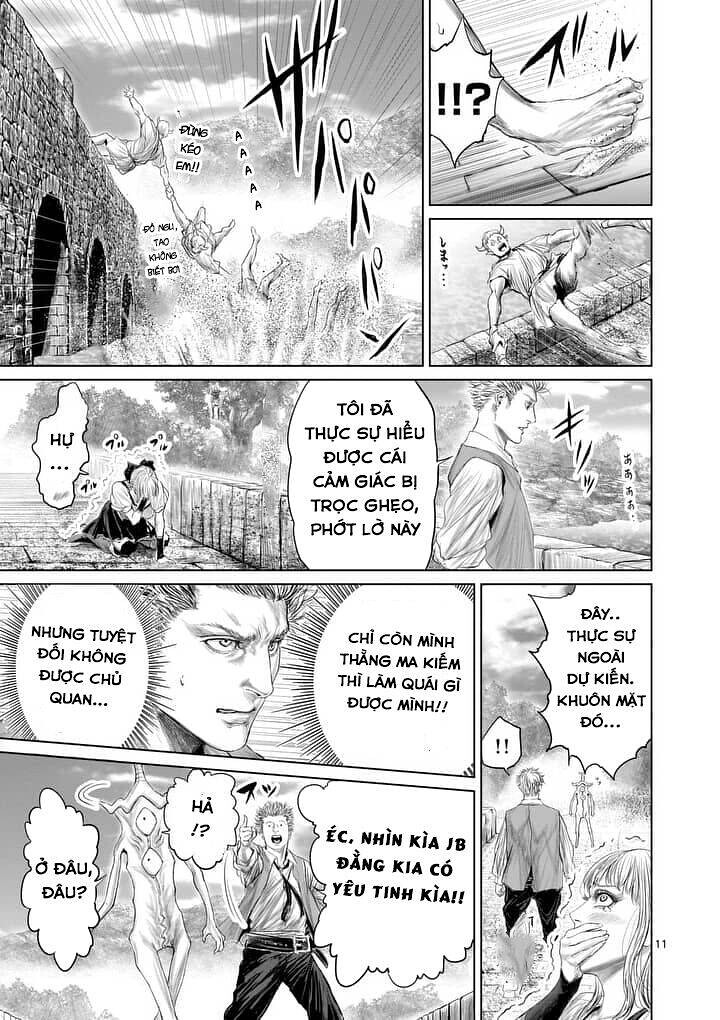The image is a black-and-white manga-style comic strip, potentially translated into Vietnamese, with its text featuring words like "Toi Da," "Tuk Su," "Hue," "Dua," "Kai," "Kam," "Chiac," "Bi," "Troc," "Gheo," "Phu," "Lo," and "Ne." The artwork is very expressive and portrays intense emotions in each scene. The comic is divided into several panels, depicting a dramatic series of events. In the initial panel, a man is slipping on a bridge while holding another person, and both are falling into water, with another individual being dragged along. Following this, a woman is shown kneeling, shaking, and crying, while observing and possibly reflecting on the situation. Suddenly, an alien or monster with two vertical eyes, resembling a walking sword, appears, intensifying the scene, with the woman scared and hiding from the creature. The detailed emotions and dynamic action sequences highlight the manga's dramatic and thrilling nature.